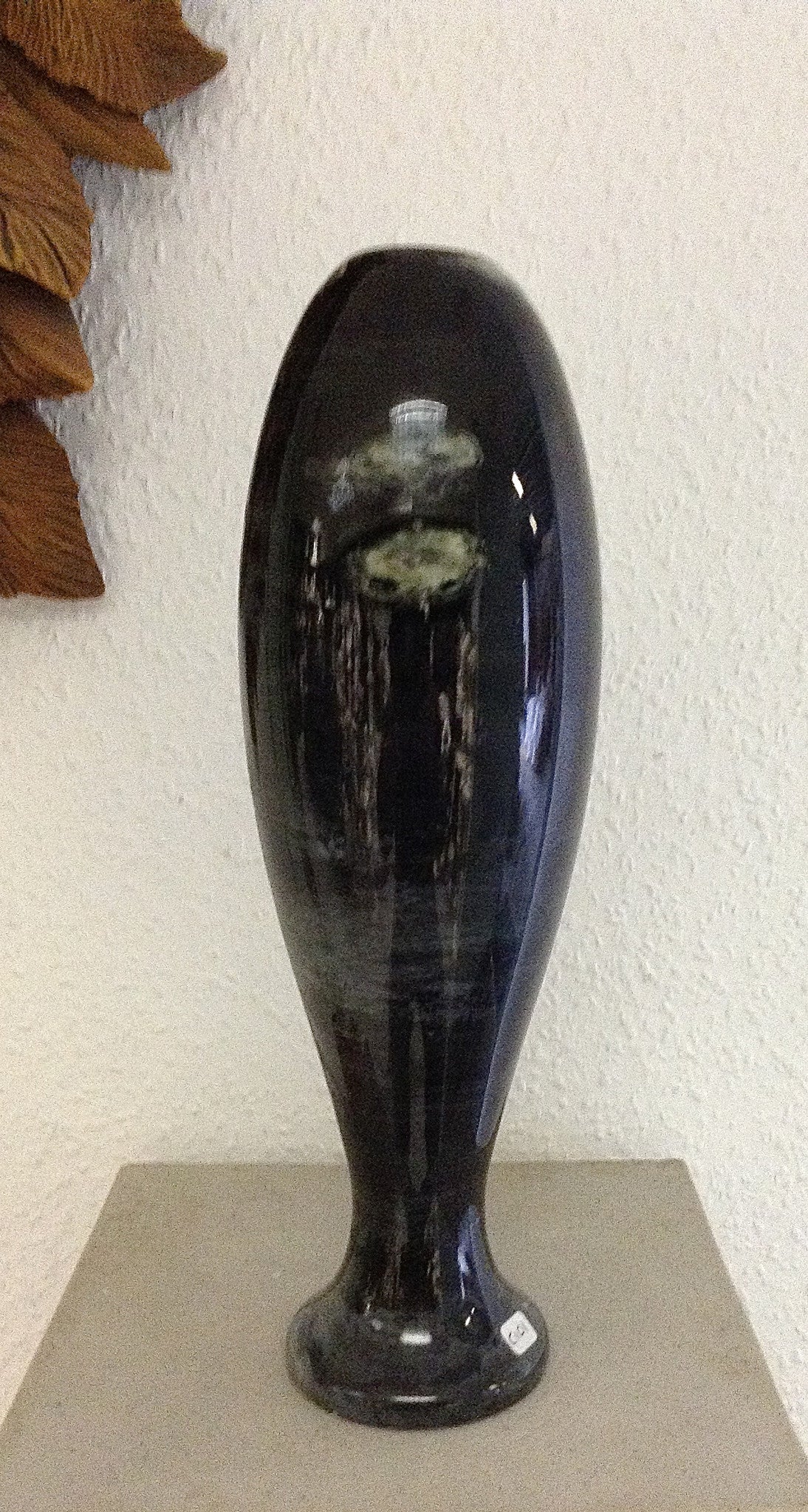This color photograph captures a candid shot of a striking art piece set against a textured white wall. The main focus of the image is a black vase-like object, seemingly upside down, with its skinnier end resting on a light gray, square-shaped pedestal. The vase tapers as it broadens towards the top, resembling a cylinder that grows more bulbous upwards. The material of the vase is slightly reflective, casting the outline of an indistinct dress or uniform across its shiny surface. To the top left of the image, a cluster of sculptural brown leaves can be seen, hinting at a wooden wall hanging. The image is devoid of any text, people, animals, or additional structures.